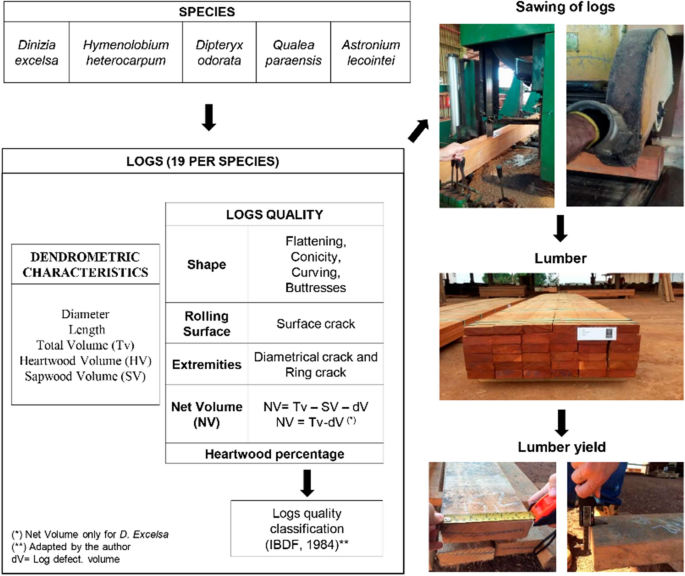The image depicts a detailed chart illustrating the lumber processing workflow, flanked by descriptive tables and step-by-step photographs. On the left, the chart begins with a labeled table listing different tree species like Denisia, Excelsa, Hymenoglobium, Heterocarpum, among others. An arrow leads to a comprehensive breakdown of log characteristics, specifying details like diameter, length, total volume, heartwood volume, and sapwood volume, in addition to log quality factors such as shape, surface, and extremities. This section is captioned "Logs, 19 per species," with an emphasis on dendrometric characteristics and quality classification.

The right-hand side showcases a series of sequential photographs visually detailing the lumber processing stages. The initial set of images displays raw logs and wood being processed by machinery. The subsequent photographs show these logs meticulously cut, polished, and neatly stacked in the field. The final images focus on close-up measurements of the finished logs, highlighting both width and additional dimensional assessments. Arrows guide the viewer through each stage, from species identification and log characteristics to the final processed lumber yield, illustrating a clear and thorough description of the entire lumber workflow.